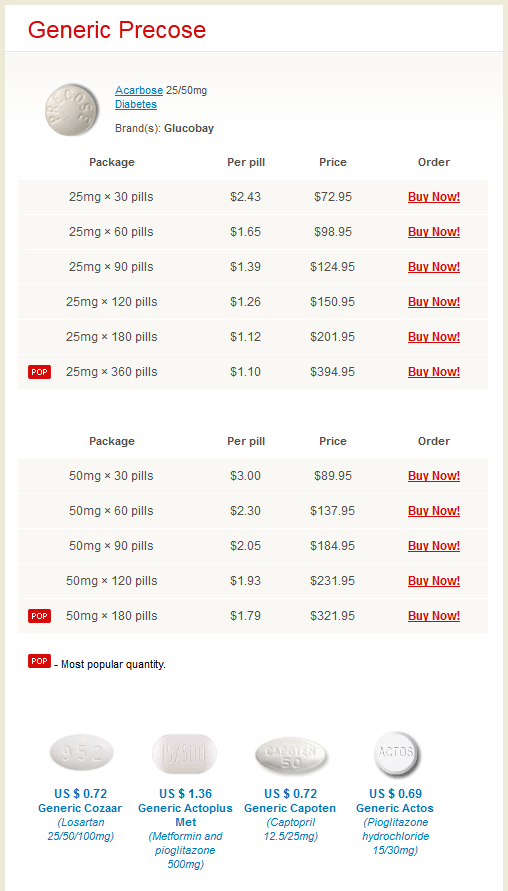This image appears to be a screenshot from a mobile device, likely an Android phone, though the specific UI elements are not visible at the top or bottom. At the top of the screen, there is a header labeled "Precalls" in bold red text with a thin separating line beneath it. Below this header, there is a section detailing a medication named "Acarbose," specifically available in 25 mg doses. The medication is indicated for diabetes treatment.

The next section is organized into multiple columns labeled "Package," "Per Pill Price," and "Order." This section lists various quantities of the medication, ranging from 30 pills to 360 pills, with prices and order options available. Each quantity option is displayed in a red, bold, and underlined font.

Following this section, there is a highlighted area marked as "Most Popular Quantity." This area lists commonly purchased quantities of the medication along with their respective per pill prices and descriptions. Each quantity option is clearly laid out, providing essential information for potential buyers.